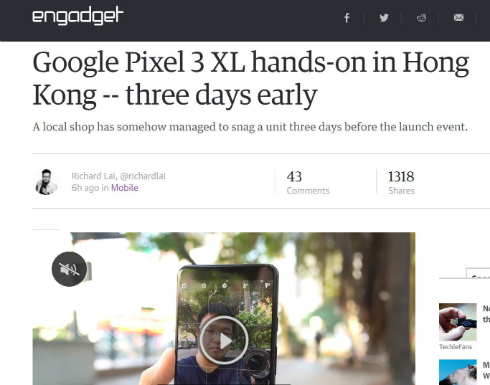The image depicts a smartphone screen displaying the Engadget website. Engadget is spelled in lowercase letters "e-n-g-a-d-g-e-t" and is positioned within a black rectangular banner at the top of the screen. This banner also contains icons for Facebook, Twitter, Google Mail, and a clock, aligned on the right side.

Below the banner, an article headline reads, "Google Pixel 3 XL hands-on in Hong Kong -- three days early." The subheadline explains, "A local shop has somehow managed to snag a unit three days before the launch event." The article is authored by Richard Lai and was published six hours ago under the 'mobile' category. Viewer interaction statistics reveal that the article has 43 comments and 1,318 shares.

Additionally, a notification bell icon, located towards the bottom, has a line through it, indicating that notifications are turned off. Centrally in the image, there is a prominent video thumbnail showing someone holding a cell phone, with a 'play' button superimposed, inviting users to view the video related to the article.